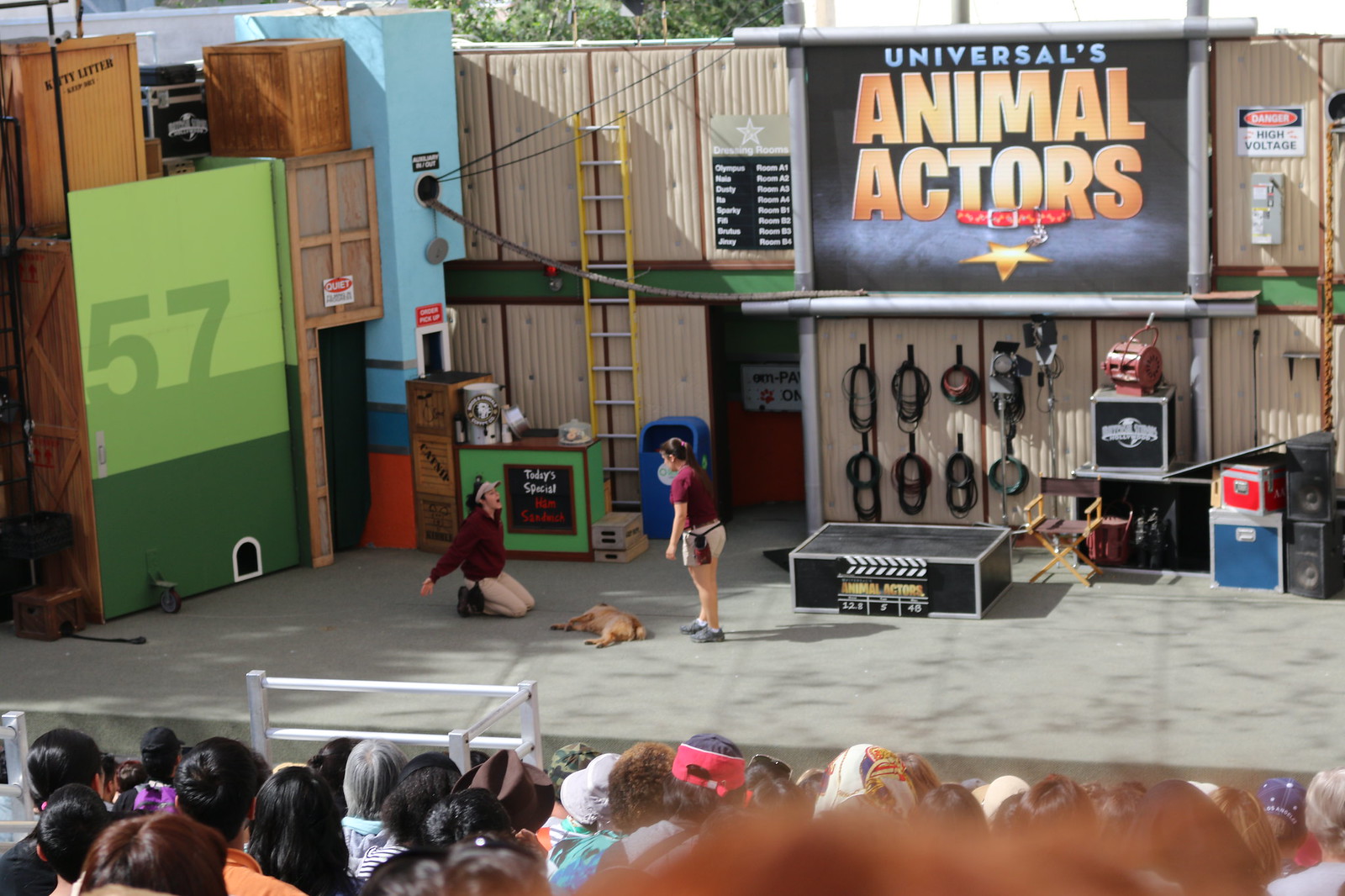The photo captures an outdoor performance at Universal Studios in their "Animal Actors" show. Taken from within a large crowd seated in an outdoor amphitheater, the image showcases a set with a concrete floor and numerous props, resembling a backstage movie set, complete with cables, boxes, crates labeled “kitty litter” and “ham sandwich,” along with a “danger high voltage” sign on a fence at the back. The backdrop, a metal wall facade, prominently displays a sign reading "Universal’s Animal Actors" in large yellow letters, and features various props including a director's chair and movie clapboard.

On stage, two young women dressed in maroon shirts and tan pants focus attention on a dog lying on its side, presumably one of the featured animal actors. The woman on her knees appears to be acting out a scene of distress over the dog, while the other stands nearby observing her. The engaging performance, highlighted by the thematic set elements like the electric equipment and labeled crates, provides a vivid behind-the-scenes glimpse into how animals are used in cinematic productions, creating an immersive and entertaining experience for the audience.